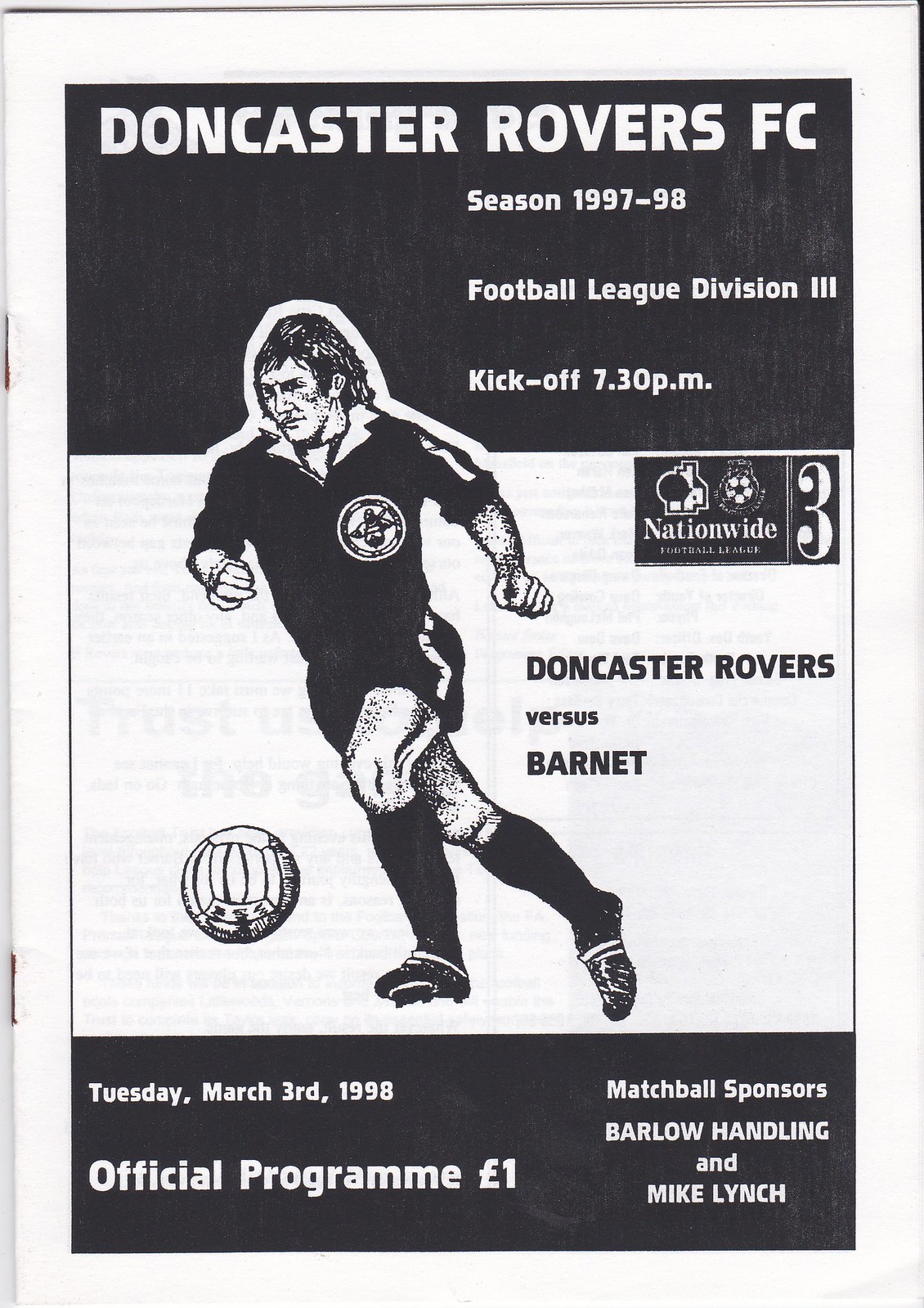This image is a black and white flyer or poster for a soccer match, likely originating from a magazine or newspaper for the 1997-98 Football League Division 3 season. It prominently features a black banner at the top with white text that reads, "Doncaster Rovers FC, Season 1997-98, Football League Division 3, Kickoff 7.30pm." Beneath this, the word "Nationwide" is showcased in a black rectangle. The center of the poster includes an illustration of a soccer player in mid-run, dressed in a jersey, shorts, socks, and cleats, poised to kick a ball. To the right of the player, the text reads, "Doncaster Rovers vs. Barnett." 

The lower section of the flyer, also with a black background and white text, indicates the details: "Tuesday, March 3rd, 1998, official program, one pound." Additionally, it mentions the match ball sponsors as "Barlow Handling & Mike Lynch." Given its layout and details, this piece likely served as an informative handout or program for attendees of the match.